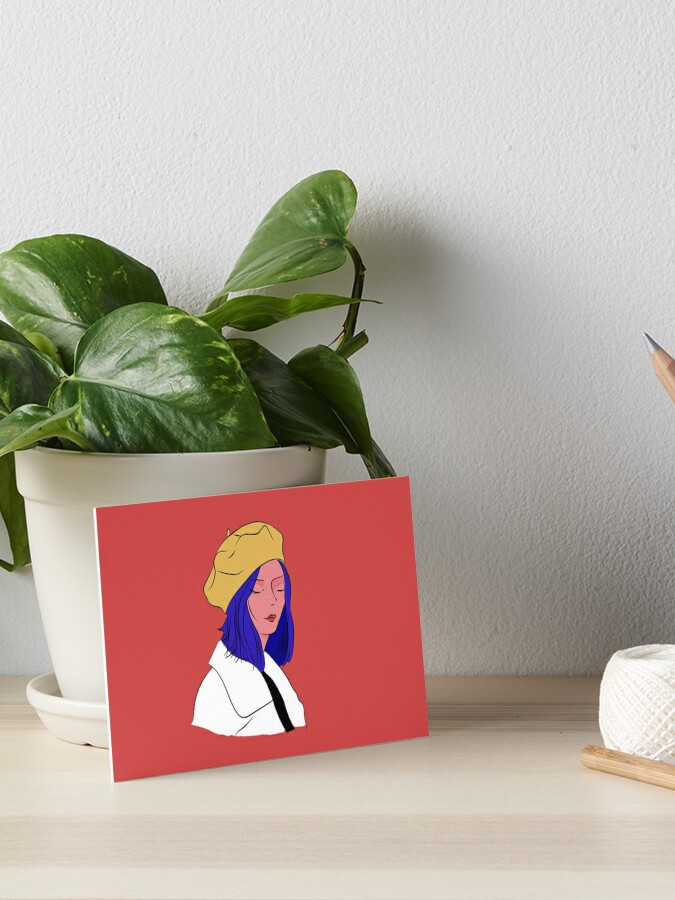The image depicts a serene, thoughtfully arranged scene on a light brown, almost natural, wooden or veneer countertop beneath a solid white wall. In the far left corner, a small leafy plant in a white pot with a matching water tray brims with vibrant green foliage, setting a fresh and lively tone. Leaning diagonally against this pot is a striking, red-background piece of artwork the size of a small thank you card depicting a woman in a black shirt and a white collared coat. The woman has dark blue hair under a tan hat, and her eyes are closed as she looks contemplatively to the right. To the right of this setup, a wooden stand holds an intricately woven ball of white twine, adding a rustic touch. Just protruding into the scene from the center right is the sharpened tip of a pencil, pointing upward and to the left, completing the composition with a hint of artistic creation.